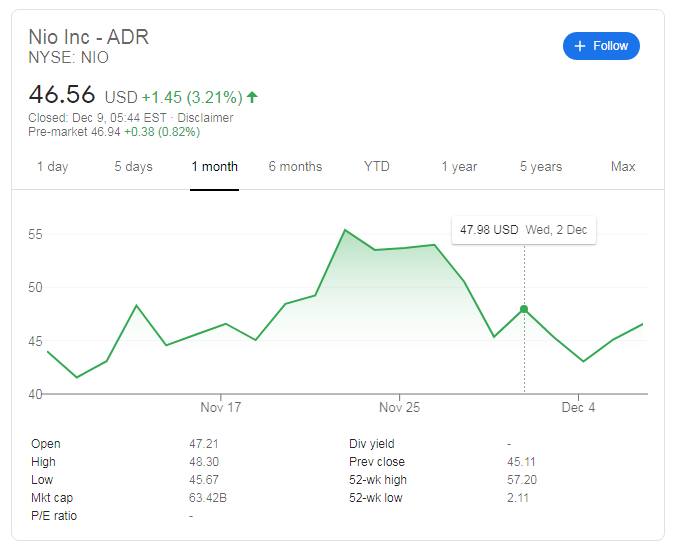The image depicts a stock app interface on a white background. In the top left section, black text and green numbers are displayed within a gray-bordered box. At the top of the box, it reads "NIO Inc - ADR NYSE: NIO." Directly below, the current stock price is shown as $46.56 USD, with a green upward arrow indicating an increase of $1.45 or 3.21%. The closing time is noted as December 9th at 5:54 PM Eastern Time. Additionally, pre-market data shows a price of $46.94, reflecting a rise of $0.38 or 0.82%.

Below this data, there are tabs for different time periods: 1 day, 5 days, 1 month, 6 months, year-to-date, 1 year, 5 years, and max. A blue "Follow" button is positioned in the upper right corner. Beneath the time period tabs, a graph visualizes the stock's performance over time.

At the bottom of the page, there are four columns providing further detailed information.